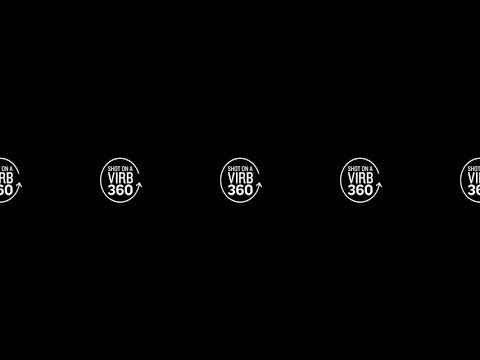The image features an entirely black background with a repeating pattern of a distinct logo and text. The logo, centrally positioned, is a white circular shape with an arrow on the right middle part, giving the impression of the circle chasing its own tail. Inside the circle, the text "SHOT ON A" appears in small capital letters on the top line, followed by "VIRB" in much larger capital letters and "360" below it, also in large capital letters. This pattern is replicated five times across the image, with the central three logos fully visible and the outer two half-visible, cut off at the edges of the image, thus emphasizing the repetition.